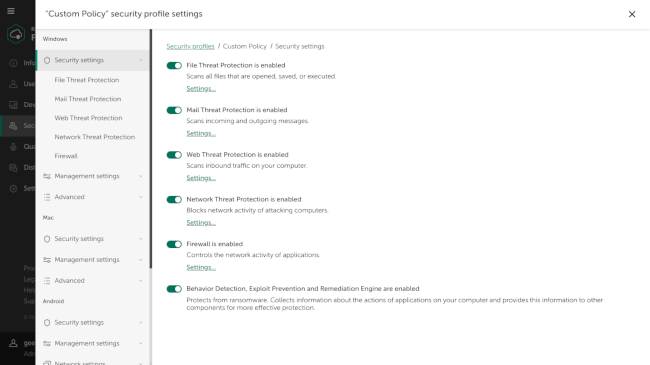The image depicts a security settings interface on a website, with no visible URL. The main view is centered around a section titled "Custom Policy Security Profile Settings" shown in a highlighted search bar. On the left-hand side, there is a navigation panel with several categories, and "Windows Security Settings" is prominently highlighted.

Below this section, individual security features are listed:
- File Threat Protection
- Mail Threat Protection
- Web Threat Protection
- Network Threat Protection
- Firewall
- Management Settings
- Advanced

Additionally, security settings for different operating systems are outlined, such as Mac and Android security settings, all grouped under section headers like "Security Settings" and "Management Settings."

The detailed security profile settings opened on the right reveal the following, all marked as enabled:
- **File Threat Protection**: Scans all files upon opening, saving, and execution.
- **Mail Threat Protection**: Scans all incoming and outgoing emails.
- **Web Threat Protection**: Monitors and scans all incoming web traffic.
- **Network Threat Protection**: Blocks suspect network activity from potential attackers.
- **Firewall**: Controls and regulates network activity of all applications.
- **Behavior Detection**
- **Exploit Prevention**
- **Remediation Engine**

Each of these security features is configured to enhance the protective measures, ensuring comprehensive threat detection and prevention across the system.